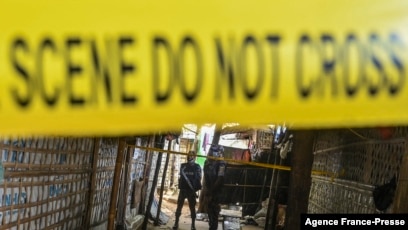This small, horizontal, close-up image captures a daytime crime scene marked by a prominent, out-of-focus yellow tape at the top that reads "SCENE DO NOT CROSS" in black letters. Below the tape, at the bottom of the image, there is also a mention of "agents France press PR ESSE." The scene reveals what appears to be the entrance to a building or alley, partially framed by walls that resemble woven sticks or cardboard. Standing beside one of these walls is a person who seems to be in a military outfit or a blue vest with a white stripe, possibly guarding the entrance. A second yellow ribbon is visible in the background. The composition suggests an environment that's open to the outside, with an open sunlit area faintly visible behind the person.